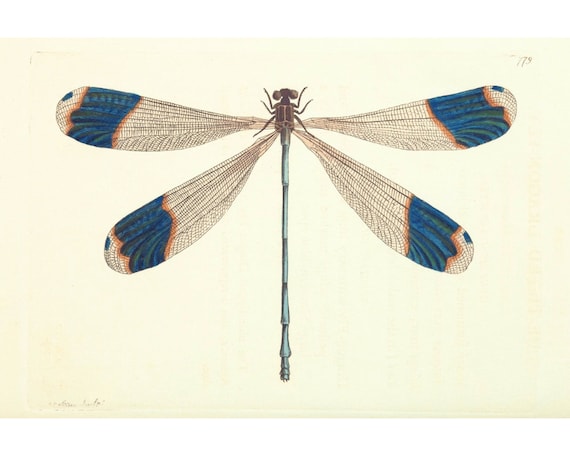The image is a detailed color drawing of a dragonfly with an elongated, segmented body, positioned centrally against a yellowish-tan background. The dragonfly's thorax is brown and adorned with six small, brown legs—three on each side. Its tail, a prominent feature, extends gracefully and is painted in a turquoise blue hue, resembling segmented bamboo. The insect's head comprises two tiny circles attached to the narrow body.

Four overlong wings, transparent and intricately detailed with thin brown or black lines, extend symmetrically from the body. These wings feature delicate netting patterns and end in sections highlighting different shades of blue bordered by striking orange stripes. The upper pair of wings extends horizontally while the lower pair angles downward gracefully. The intricate artistry of the wings includes curved gray and green stripes towards their tips. The overall effect is a meticulously detailed and vibrant representation of a dragonfly in flight.